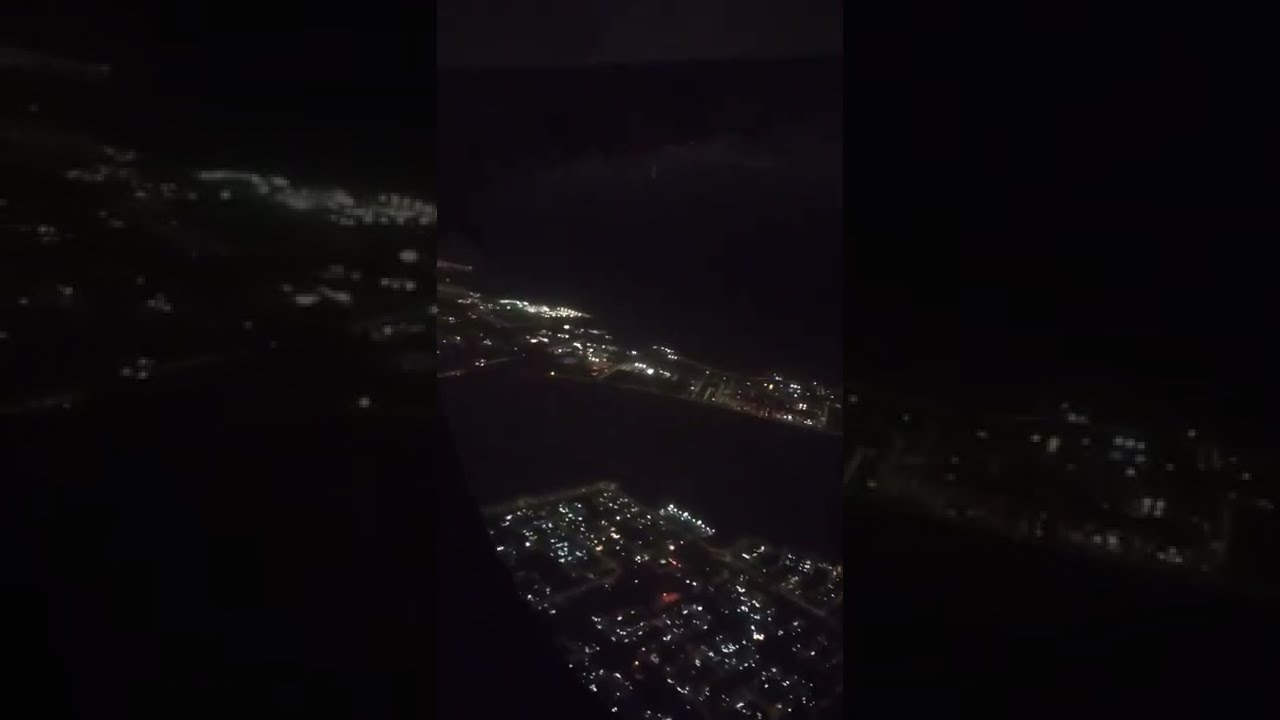This image, rectangular in shape and measuring about six inches wide by four inches tall, appears to be an aerial shot taken from an airplane or cockpit, looking down at a nightscape. The scene is divided into three distinct sections: left, center, and right. The central section showcases two illuminated strips of cityscape, one running horizontally with bright lights suggesting streets or buildings. These strips are interspersed with dark areas likely representing water, creating the appearance of islands divided by black stretches of water. The sky above is completely black, with some gray clouds visible, adding to the nighttime ambiance. On the left and right sections of the image, there are enlarged and darkened views of portions of this land, with the left appearing blurrier in contrast to the clearer central strip. The lights in the center show dots of reds and whites, hinting at the lively and bustling nature of the city below.